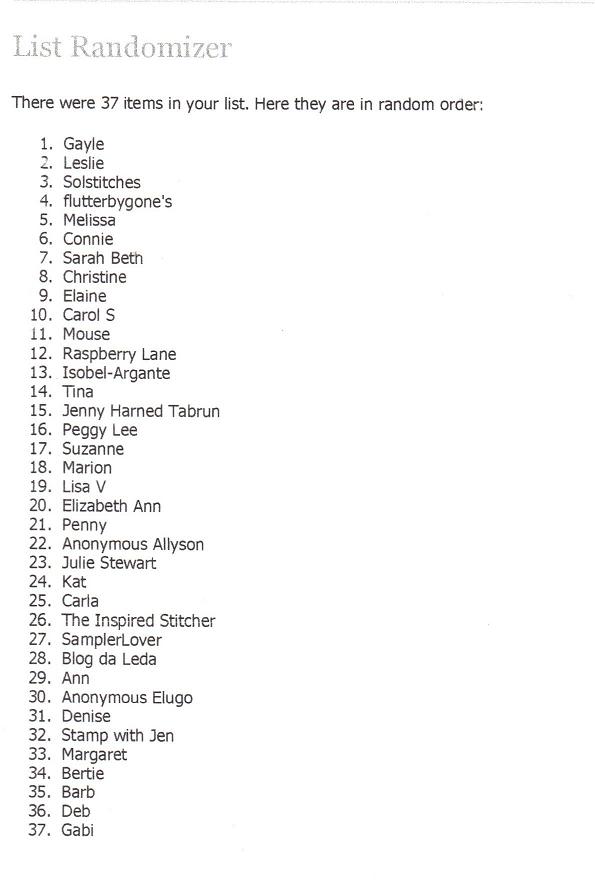In the image, a printed or digital list is captured prominently. The header, written in a larger font, states "List Randomizer." Below, it mentions, "There were 37 items in your list. Here they are in random order:" followed by a colon. The list beneath this heading is numbered sequentially from 1 to 37 on the left-hand side, accompanied by corresponding names or terms aligned on the right.

At the very top, the number 1 position reads "Gail." The subsequent entries follow in order: 

2. Leslie
3. Soul Stitches
4. Flutter By Gons
5. Melissa
6. Connie
7. Sarah Beth
8. Christine
9. Elaine
10. Carol S
11. Mouse
12. Raspberry Lane
13. Isabel Agente
14. Tina
15. Jenny Harned Tabon
16. Peggy Lee
17. Suzanne
18. Marion
19. Lisa V
20. Elizabeth
21. Penny
22. Anonymous Allison
23. Julie Stewart

The list continues similarly down to:

31. Gabby

The photograph clearly represents a randomized assortment of items, each distinctively listed with their positions reshuffled.